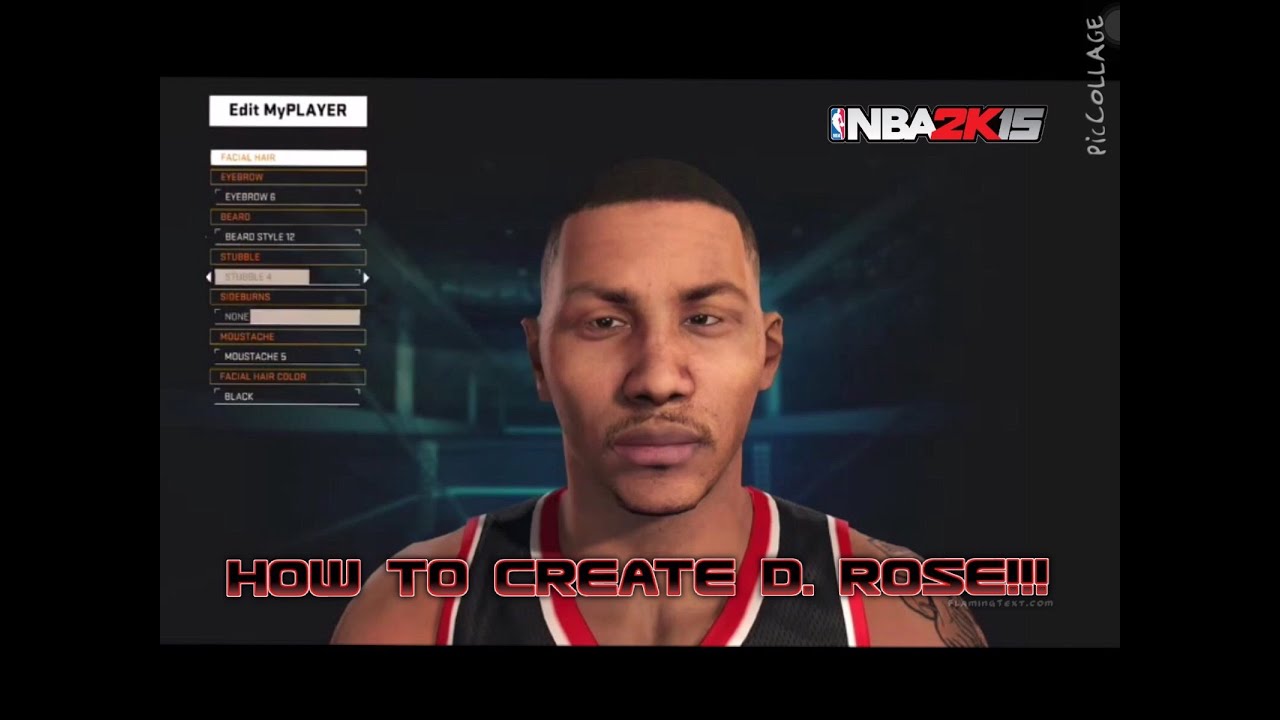A detailed representation of a video game character creation screen can be seen in the image. The background depicts a stadium-like atmosphere, suggesting the setting of a sports arena. On the right side of the screen, there's a section labeled "Pie Collage," alongside the title "NBA 2K15." Further down, the option "Edit My Player" is visible, indicating the customization features available for the character.

The character being customized is a man with short black hair and notable facial details. His facial hair includes neatly groomed eyebrows, a 12-day stubble along the jawline, and a light mustache. His complexion reveals slight wrinkles on his forehead, giving him a more mature appearance. His lips are pinkish in tone.

The character is dressed in a black jersey vest, accented with white and red stripes, signifying a sporty look possibly aligned with a basketball team. He also has a tattoo on his arm, adding to his personalized and unique appearance.

Additionally, the interface includes various customization options, such as facial hair styles and color settings indicated by "stubble" and "hair color black." There is also an instructional or promotional text reading: "How to create the rose," potentially referring to a specific customization feature or tool. 

Overall, this image encapsulates the immersive and detailed character customization available in the NBA 2K15 video game, allowing users to create their personalized players with extensive options.